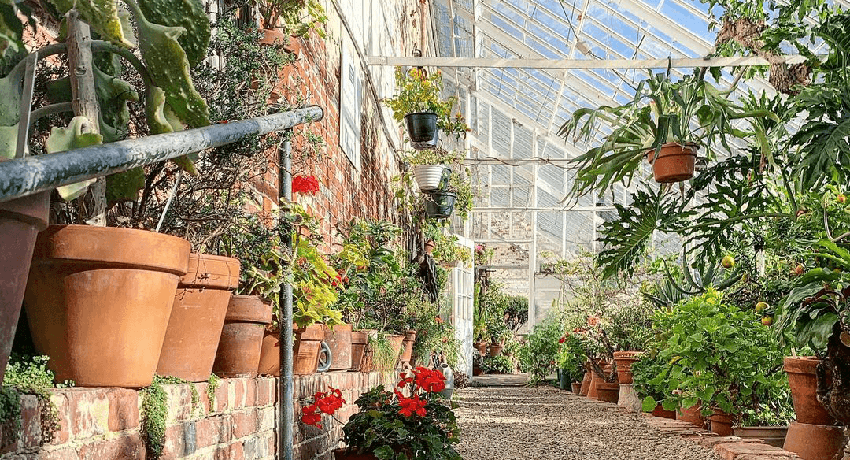This image captures the interior of a verdant greenhouse characterized by a variety of lush plants. The greenhouse features a distinct slanted roof, allowing ample sunlight to filter through and nourish the greenery within. The walkway, fashioned from stone, runs centrally through the space, with the left and right sides densely packed with botanical beauty.

On the right side, an assortment of plants is neatly arranged atop a brick ledge. Some of these plants boast thick foliage and long stalks, creating a rich tapestry of greens. Hanging from the ceiling are more plants, cascading elegantly over their pots. Among these, one particularly eye-catching plant with bright red flowers stands in front of the brick wall, adding a vibrant splash of color to the scene. An iron railing ascends from the center of this area, indicating steps, which add a dynamic architectural element to the greenhouse.

The left side of the greenhouse is equally abundant with flora, featuring striking long-leaved plants that drape downward in a spider-like fashion. Interspersed among these are plants bearing fruit, possibly pears, contributing to the diversity of the greenhouse's collection. This side is lined with numerous potted plants that extend along the gravel path, which gently guides the viewer's gaze to an open door. This door hints at another room within the greenhouse, inviting curiosity and promising further horticultural delights beyond the frame of the picture.